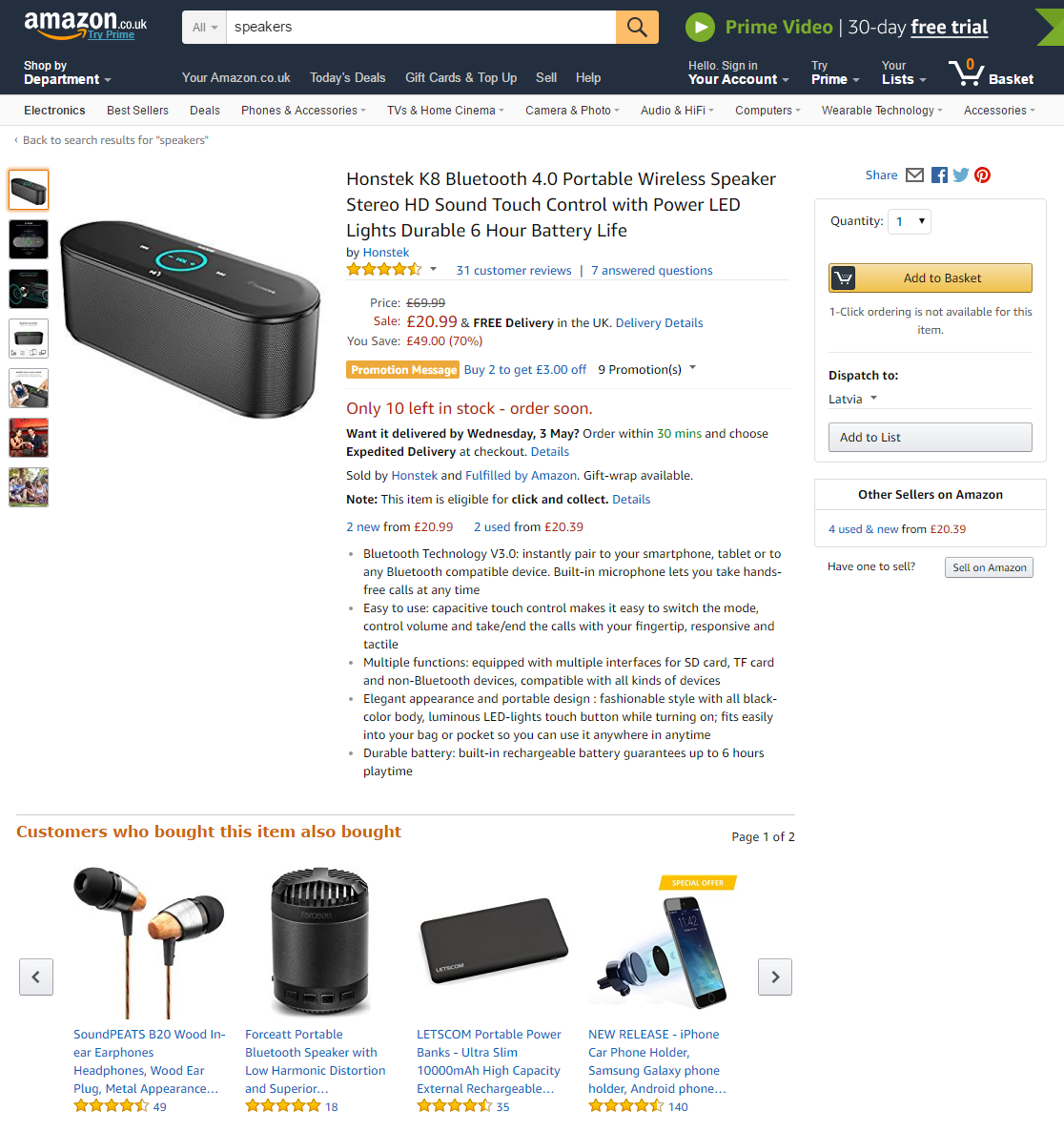In the image, an Amazon page is prominently displayed. At the top center of the page, the Amazon logo is clearly visible. Directly to the right of the logo, there's a search bar with a magnifying glass icon on its right side, distinguished by its orange background. The left part of the search bar is white and contains the text "Speakers."

To the right of the search bar, a green arrow within a circle accompanies the text "Prime Video," followed by a note indicating a "30-day free trial." Below this strip are various navigation options, including links to "Your Account," "Prime," "Your Lists," and "Your Shopping Cart," which is labeled as "Your Basket" on this platform.

Beneath these options, there is a list of ten categories: Electronics, Best Sellers, Deals, Phones and Accessories, TVs and Home Cinema, Carriers and Photo, Audio, Computers, Wearable Technology, and Accessories.

The main product showcased on the page is a "Hansek K8 Bluetooth 4.0 Portable Wireless Speaker." This speaker features HD sound, touch control with power LED lights, and a durable battery life of 6 hours. The text describing the product is in black, and the price is listed as $20.99.

Further down the page, there is a section titled "Customers Who Bought This Item Also Bought" in orange text. In this section, four related items are displayed. On the right-hand side of the product listing, there is an "Add to Basket" button, with the quantity set to 1, concluding the details shown in the image.